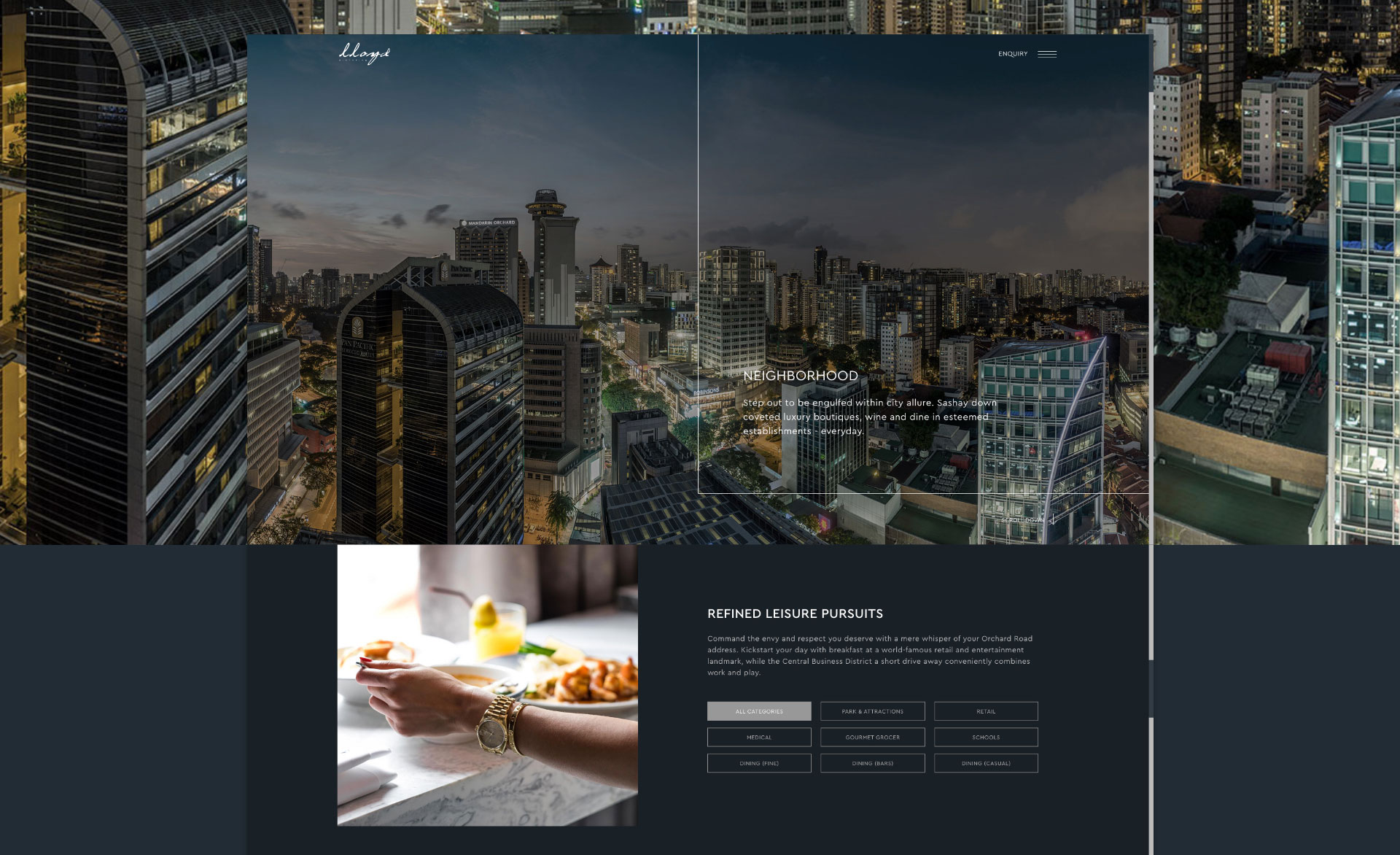A glossy brochure showcasing an upscale urban lifestyle prominently features an array of towering skyscrapers and vibrant city scenes. From a vantage point within a luxurious restaurant, diners can enjoy sweeping views of the illuminated cityscape, highlighting the diverse and striking architecture of the metropolis.

The brochure invites readers to "step out to be engulfed within city allure," encouraging them to explore high-end boutiques, and savor culinary delights at esteemed establishments daily. Complementing this text is an enticing image of gourmet food alongside a sophisticated cocktail, implying a lavish dining experience.

Additionally, the brochure notes, "command the envy and respect you deserve with a mere whisper of your Orchard Road address." It emphasizes the convenient location, suggesting that one can start their day with breakfast at a renowned retail and entertainment landmark, while the central business district, just a short drive away, seamlessly blends work and leisure.

The brochure categorizes various amenities and facilities nearby, listing options under medical, dining, attractions, gourmet grocer, dining areas, retail, schools, and casual dining. The dining options are subdivided into three tiers—budget, mid-range, and high-end—catering to a variety of tastes and preferences.